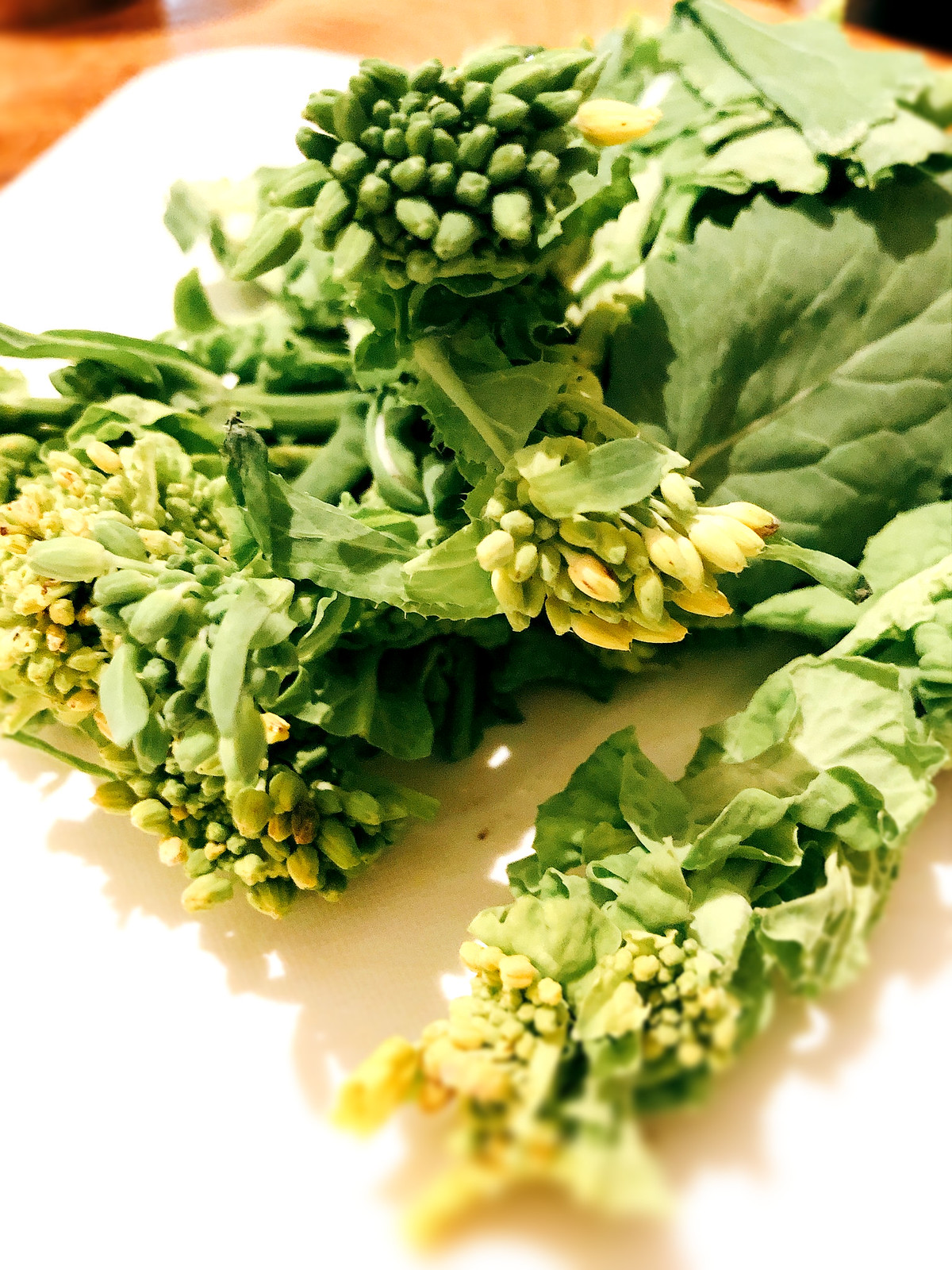This close-up image features a bunch of leafy greens, likely broccolini, organized on a square white plate, creating a striking contrast against the wooden tabletop it rests on. The plant appears to have large, deep green leaves with prominent white veins, and the tops are adorned with yellow and green buds that resemble miniature flower heads about to bloom. Some leaves and buds are casting distinct shadows under the bright artificial lighting from above, hinting at a lamp nearby. Toward the front of the image, there's some blurring, but the central focus remains clear, capturing the fine details of the leafy texture and budding tops. The white plate’s surface reflects some parts of the greens, intensifying their vibrant colors. In the background, you can spot a light beige marble countertop, adding another layer of texture, with a small portion shaded black, and the warm orangey-brown hue of the wooden table adds a homely feel to the scene.